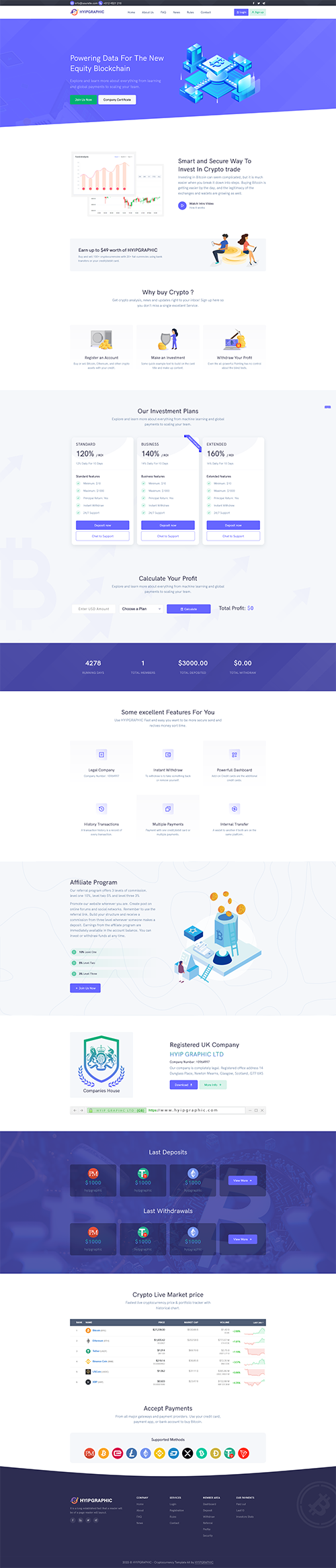This image is a vertically-oriented screenshot of a lengthy website, capturing several sections in a single frame. Due to the distance at which the screenshot was taken, the text on the website is unreadable. The top section of the first page features a blue banner, accompanied by what appears to be an illustration related to a living room display situated to the right. Below the banner, the background shifts to white, displaying various internet tabs, a graph, and illustrations of people engaged in activities on a couch. Beneath this, there is a gray section showcasing three distinct pricing options. This gray section is followed by another white background containing additional tabs and options, along with another illustration. The website's design alternates between purple and white sections throughout, creating a visually segmented layout. Despite the details evident in the design elements, the overall small scale makes specific content illegible.